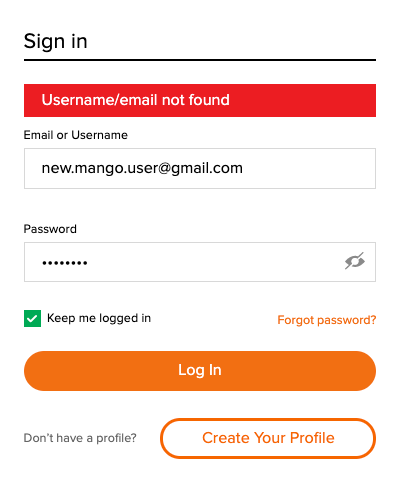The image depicts a sign-in interface displayed on a smartphone screen.

At the top, a red box appears with the error message "Username/Email not found" beneath the header "Sign-In." Below this message, an input field labeled "Email or Username" is filled with the text "new.mango.user@gmail.com." 

Directly underneath is a labeled field for "Password," which conceals the entered password as a series of dots for security. Next to this field is an eye icon with a slash through it, indicating password visibility control.

Further down, a green box with a white checkmark contains the option "Keep me logged in" in black text. Beside this is the "Forgot password" link, highlighted in an orangish-red color.

Toward the bottom of the screen, there is an orange, rounded-rectangle button with the text "Log In" in white. Below this, a gray text prompts "Don't have a profile?" followed by "Create your profile" in white and orange text, directing users to the account creation section.